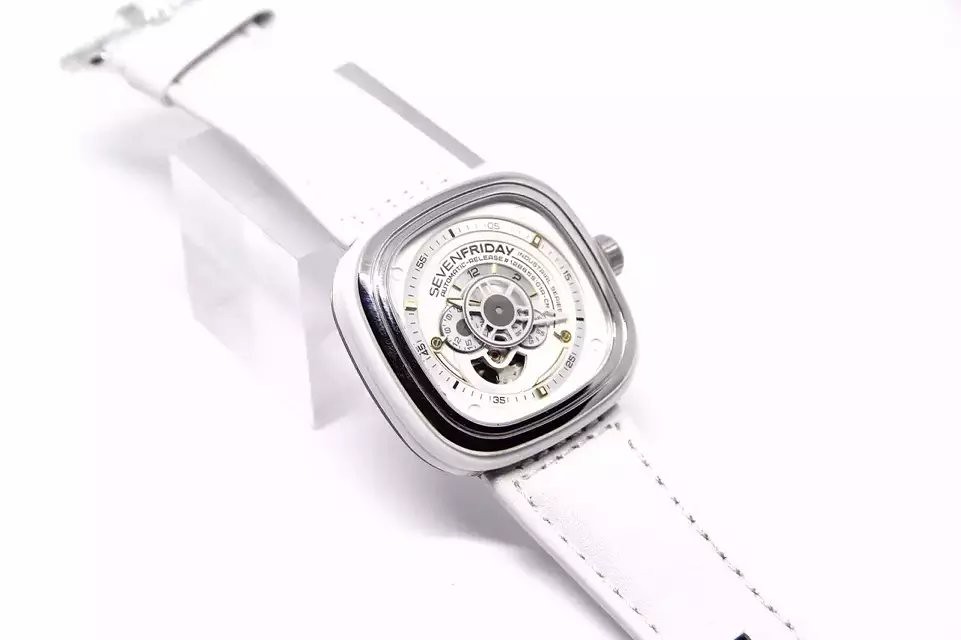This photograph showcases an elegant wristwatch positioned almost perfectly in the center of the frame. The timepiece features a uniquely styled square case in white and silver, paired with a pristine white leather strap. The watch face is intricately designed with multiple gears and dials, adding to its sophisticated appearance. A winding stem is prominently placed on the right side of the square case. One half of the leather strap is artistically draped over a translucent cube to create an angled display of the watch. Both the cube and the watch rest on an immaculate white surface, enhancing the overall aesthetic with a clean, minimalist background. Silver accents from the watch face, winding stem, and buckle on the left side add a touch of refinement to the predominantly white composition.